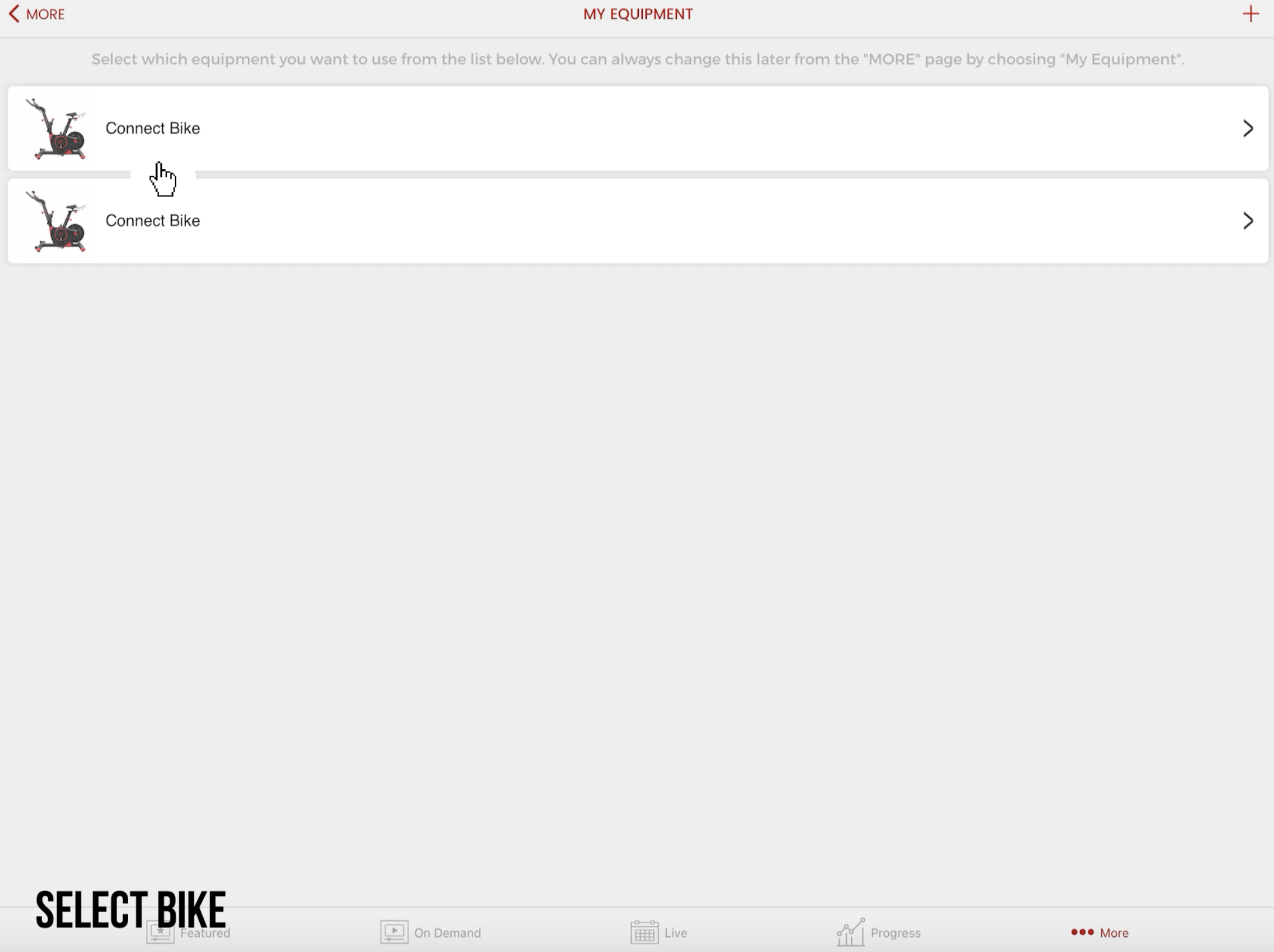The image displays a user interface for selecting and managing cycling equipment. 

The top left corner features the options "More," "My Equipment," and "Redsys Plus." Below this, a detailed instruction reads, "Select which equipment you want to use from the list below. You can always change this later from the More page by choosing My Equipment." 

A section labeled "Connect Bike" showcases a bicycle icon followed by a right arrow, indicating the option to select this bicycle. Another bicycle icon follows with the same "Connect Bike" label and right arrow.

In the bottom left, the text "Select Bike" is written in black. Adjacent to it, icons represent various features: a TV with "On Demand," a calendar labeled "Live," and a line graph with circles indicating "Progress." 

Additional navigation options are indicated by three red dots, followed by the text "More." The background is gray, suggesting this is likely the main interface for the Connect Bike application.